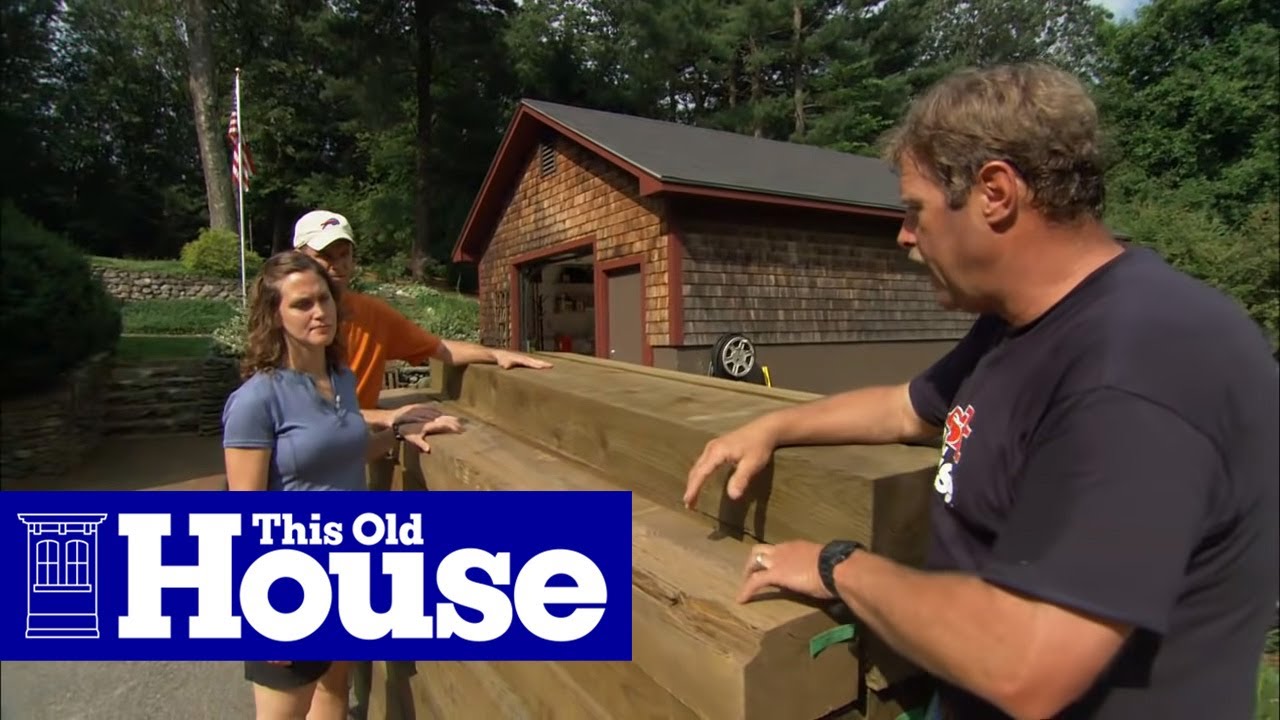This detailed image appears to be a screenshot from the reality TV show "This Old House." At the bottom left corner, there's a blue banner with the white text "This Old House," featuring small text for "This Old" and a large "H" for "House." The scene captures three individuals standing in front of a stacked pile of wood resembling bleachers. 

On the right side of the image, an older man in his fifties with gray and blonde hair, wearing a black t-shirt with red and white lettering, leans against the wood. He has a black watch and a gold ring on his wedding finger. His left arm rests on the wood while his right arm sits atop it. 

In the middle of the frame, a woman with long blonde hair is seen wearing a blue t-shirt and black shorts. Part of her arm is obscured by the "This Old House" label. She stands next to another man who is wearing an orange t-shirt and a white Buffalo Bills hat, with his left hand resting on the wood.

In the background, a lush scene unfolds with large green trees, a high flagpole with an American flag, and a well-kept lawn. There's also a garage or shed with wood trim and a black roof, which has a water hose wrapped around a holder resembling a tire attached to it.